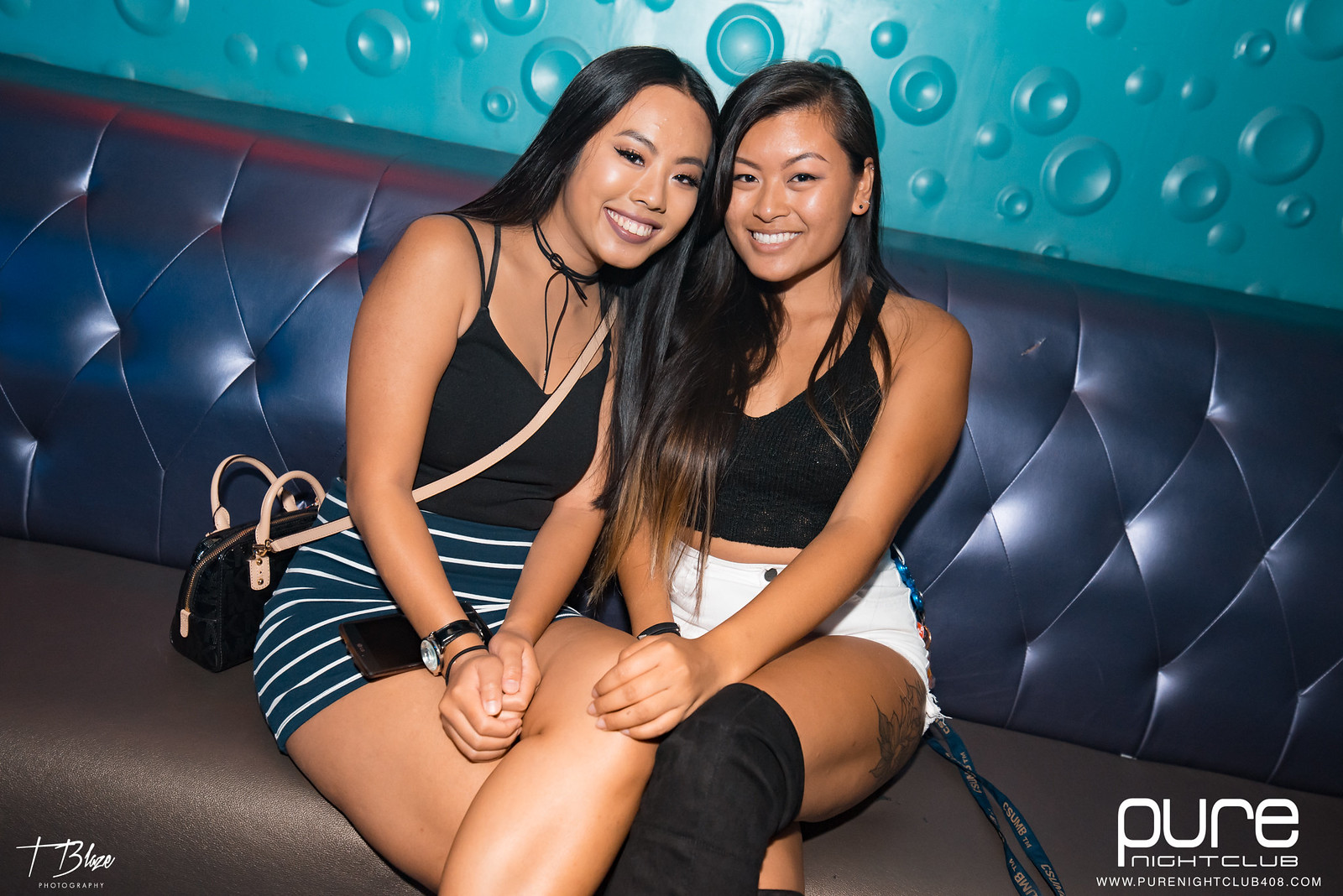In this detailed photograph of a horizontal rectangular layout, two women, appearing to be in their early to mid-20s and of Asian descent, are seated very closely together on a navy blue faux leather bench with a puffy quilted back. The backdrop is an aqua or teal-colored wall adorned with large raised circles, adding a textured appearance. Both women, smiling warmly at the camera, boast long straight hair; the woman on the right has black hair with brown tips, while the one on the left has full black hair. They both wear black spaghetti strap tank tops, exuding a casual, yet stylish vibe. The woman on the right is dressed in white blue jean shorts paired with thigh-high boots, showcasing a tattoo on her thigh, and has a lanyard dangling from her shorts. Meanwhile, the woman on the left sports a blue and white horizontal striped skirt (or possibly shorts) and wears a choker around her neck with a small purse slung over her shoulder. In the lower right corner of the image, large white letters spell "PURE," with "nightclub" beneath it, and a website link: www.purenightclub408.com. The bottom left corner bears the signature "Tea Lay's Photography," subtly crediting the photographer.